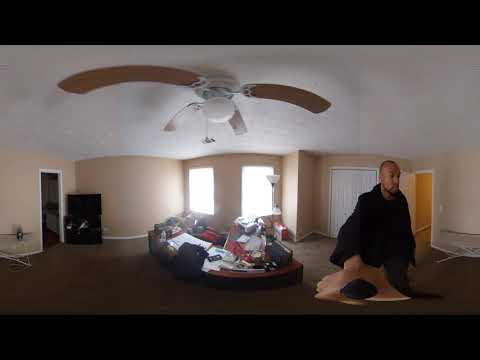This fisheye lens image captures an interior room of a house, possibly a bedroom, with a slightly distorted panoramic view, giving it a virtual reality feel. The room features a solid black border at the top and bottom, framing a carpeted floor. Dominating the center is a large, cluttered pile of various objects, resembling either a messy desk or a couch overwhelmed with clutter. Above this central chaos, two windows allow bright sunlight to filter in, illuminating the space. 

A ceiling fan with a light fixture and pull cord hangs at the top of the image, its blades appearing bent due to the fisheye effect. On the right side, a young African American man with short hair, a beard, and a mustache is present, holding a selfie stick, generating speculation on whether he is part of the image or digitally inserted. The man wears a dark coat, standing near an open double door leading into a hallway. To the left, another doorway leads into a darker room. The color palette of the image includes shades of black, white, brown, tan, gray, red, and green, contributing to the lived-in, slightly chaotic atmosphere depicted.